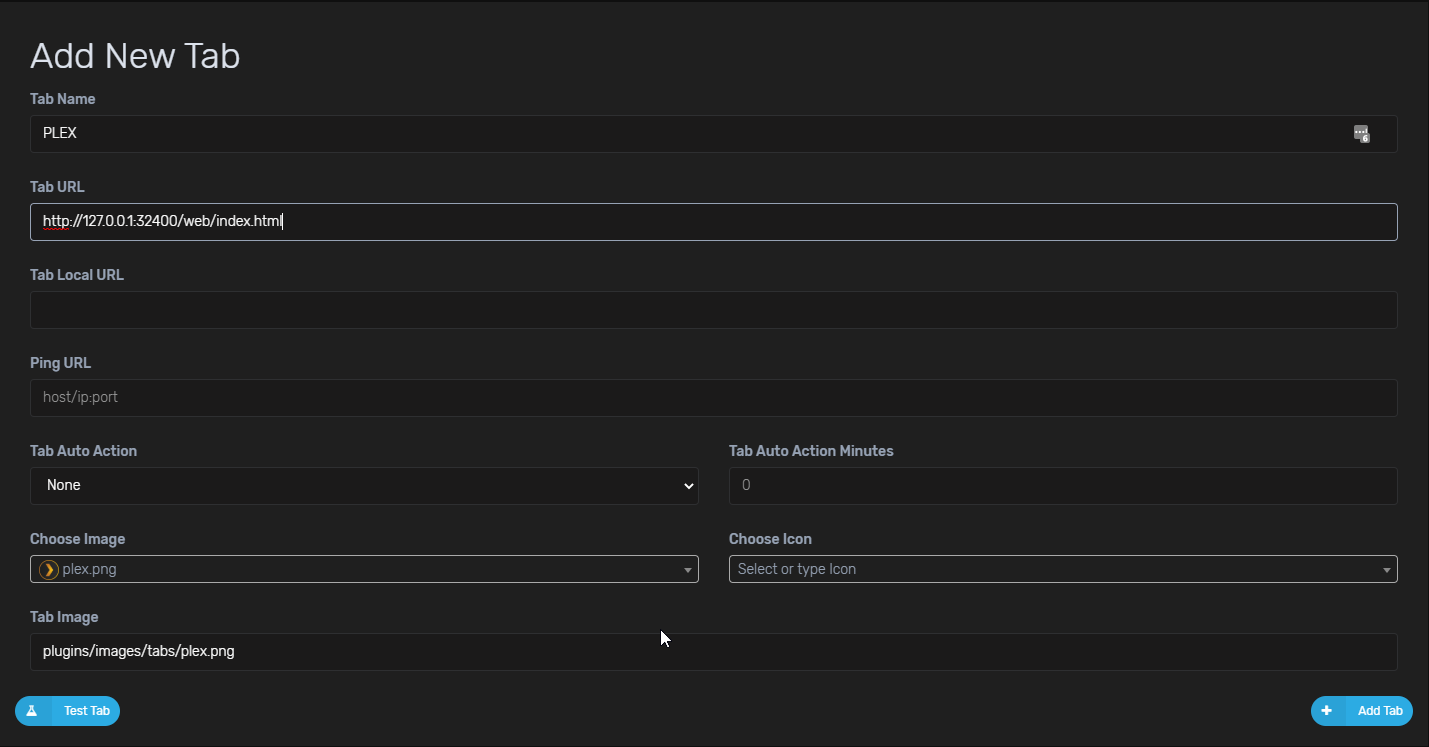The image depicts a screenshot taken either from a phone or computer screen, showcasing a dark interface with a predominantly black background. In the top corner of the screenshot, there is a section labeled "Add New Tab." Below this header, several fields and options are visible:

1. **Tab Name**: "PLEX" (written in all capital letters).
2. **Tab URL**: Displaying "http://" followed by a sequence of numbers and a web address.
3. **Tab Local URL**: The corresponding field is left empty.
4. **Ping URL**: Contains the text "host / IP.port."
5. **Tab Auto Action**: Set to "None."
6. **Tab Auto Action Minutes**: Set to "0."

Towards the lower part of the interface, there is an area titled "Choose Image." Accompanied by an orange arrow pointing right, it contains the text "Plex.png." Below this, there's another section labeled "Choose Icon" with the instruction "Select or type." Finally, at the very bottom of the screen, there is an "Add Tab" button.